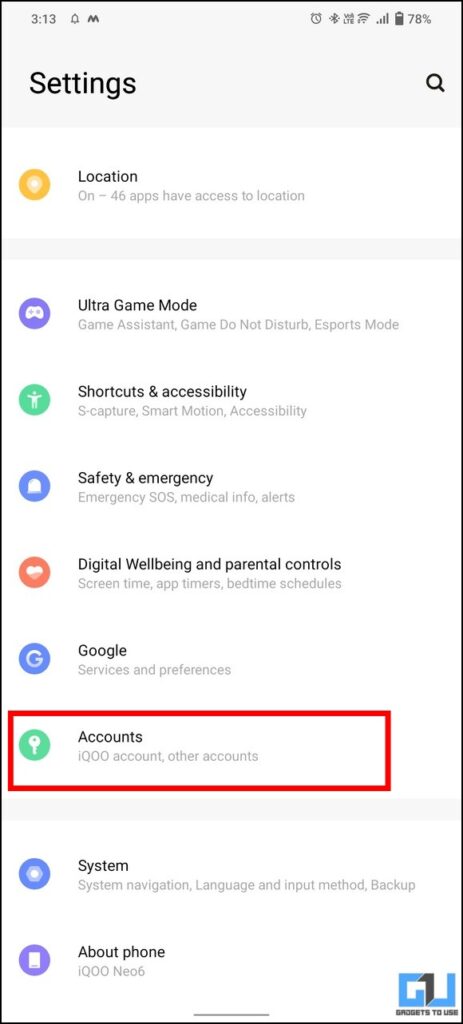The image depicts a detailed settings screen of a mobile phone, characterized by its white background and black text. At the very top left of the screen, the time is displayed as "3:13" in black text, while the right side shows several icons including a bell, clock, LTE indicator, WiFi signal, and a battery percentage at 78%. The title "Settings" is highlighted on a light grey background next to a search button.

Below the title, several settings categories are listed:

1. **Location**:
   - Description: "All 4 to 6 apps have access to location."
   - Icon: An orange or yellow circle with a white location marker inside.

2. **Ultra Game Mode**:
   - Sub-options: Game Assistant, Game Do Not Disturb, eSports Mode.
   - Icon: A bluish-purple circle with an eye mask icon inside.

3. **Shortcuts & Accessibility**:
   - Options: Accessibility features, S Capture, Smart Motion.
   - Icon: A circle containing a person silhouette.

4. **Safety and Emergency**:
   - Features: Emergency SOS, Medical Info Alerts.
   - Icon: A highly blurred image, but possibly resembling a bed or tombstone.

5. **Digital Wellbeing and Parental Controls**:
   - Tools: Screen Time, App Timers, Bedtime Schedules.
   - Icon: A small circle with what appears to be a heart.

6. **Google Services and Preferences**:
   - Icon: A blue "G" symbolizing Google.

7. **Accounts**:
   - Details: i000 account, other accounts.
   - Icon: A green circle featuring a key.

The "Accounts" section also has a superimposed red box outline.

8. **System**:
   - Options: System Navigation, Language and Input Method, Backup.
   - Icon: A blue round thingy.

9. **About Phone**:
   - Information: I000 NEO6.
   - Icon: A purple circle with a white phone icon.

At the very bottom of the screen, a thin black bar spans across roughly one-fifth of the page. To the lower left, there is a faint watermark that appears to read "Gadgets to USA" in blue and black text, indicating the potential source of the screenshot.